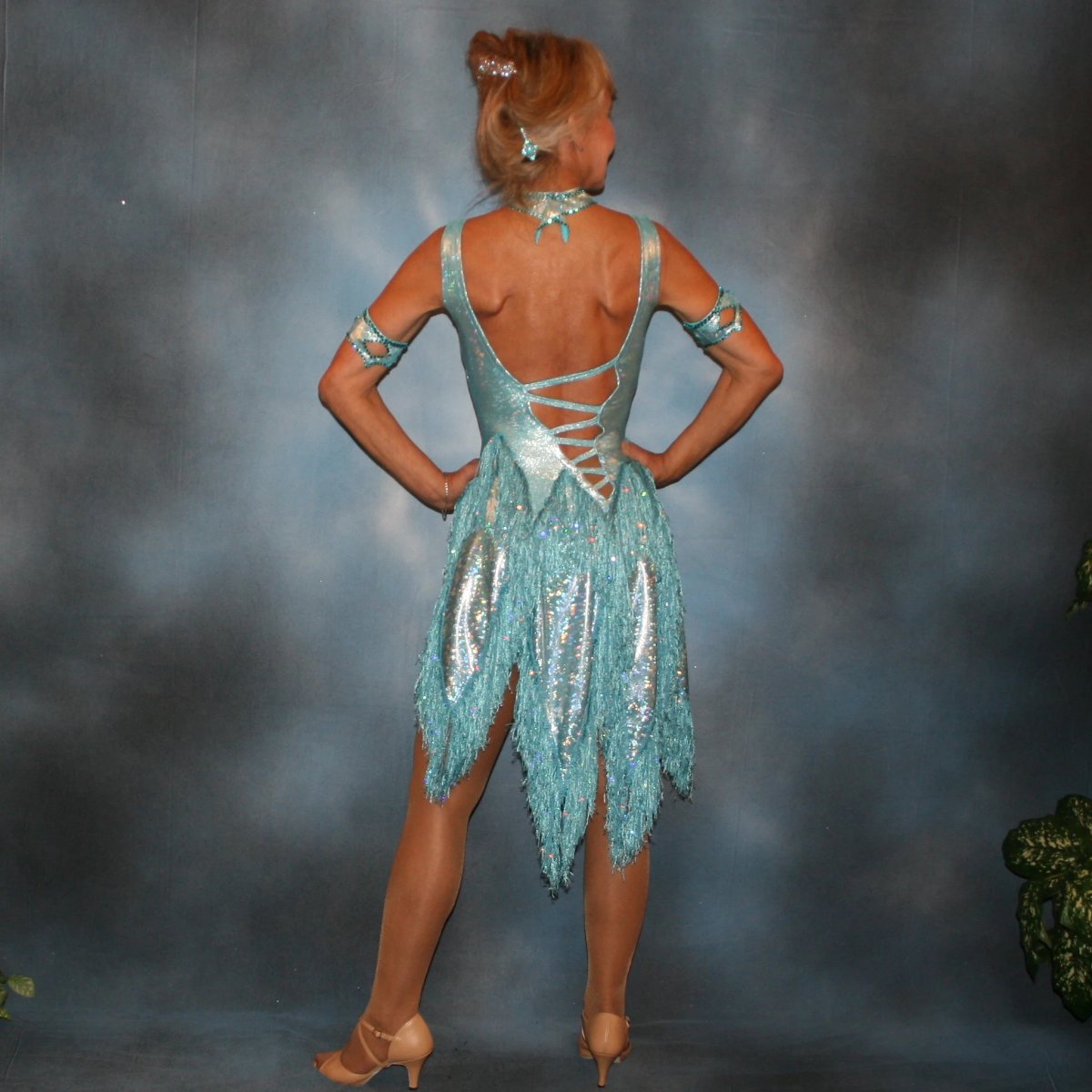The image depicts a woman standing with her back to the viewer in front of a faded, blue-and-white background, resembling a studio photo setting. She is dressed in an elaborate, shiny, metallic light turquoise costume that suggests she might be a dancer or showgirl. Her outfit features an asymmetrical dress with a handkerchief hem and fringe, incorporating several panels of metallic fabric. The back of the dress forms a V that points to the right, leaving much of her back exposed except for straps along the sides. She wears cut-out upper arm bands, jeweled pins in her updo, and a choker fastened from the back, all matching the light turquoise theme, adding to the cohesive metallic look. Her tan three-inch high heels, ribbon-tied choker, and hands resting on her hips complete the poised stance as she slightly turns her head to the right, showing glimpses of her hairstyle adorned with glittering barrettes.